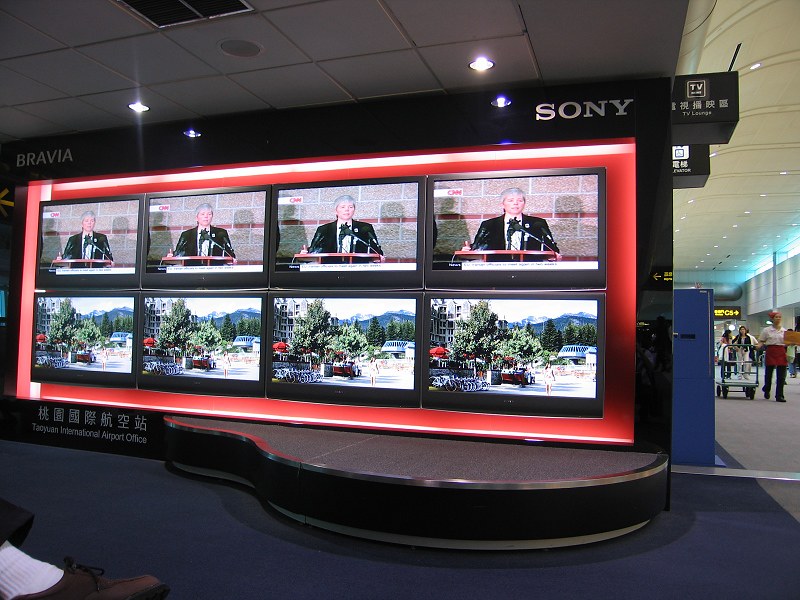The image depicts a section of Taoyuan International Airport, specifically within an area labeled as the "TV Lounge." It prominently features a large red-framed display composed of eight flat-screen televisions arranged in two rows of four. The top row of screens shows an image of a woman speaking at a podium with a CNN logo, while the bottom row displays a scenic view of a road bordered by parked bicycles, trees, and a building, with what appears to be a mountain range in the background. Above the televisions, the left side is branded with the Bravia logo and the right side with the Sony logo. In the foreground, there is a circular black plinth in front of a dark blue carpeted floor, and a brown shoe with a white sock is visible at the bottom left corner. To the right of the display, a gangway reveals several people, some appearing to shop or walk towards their gates, with one individual wearing a red apron and pushing a silver dolly cart.